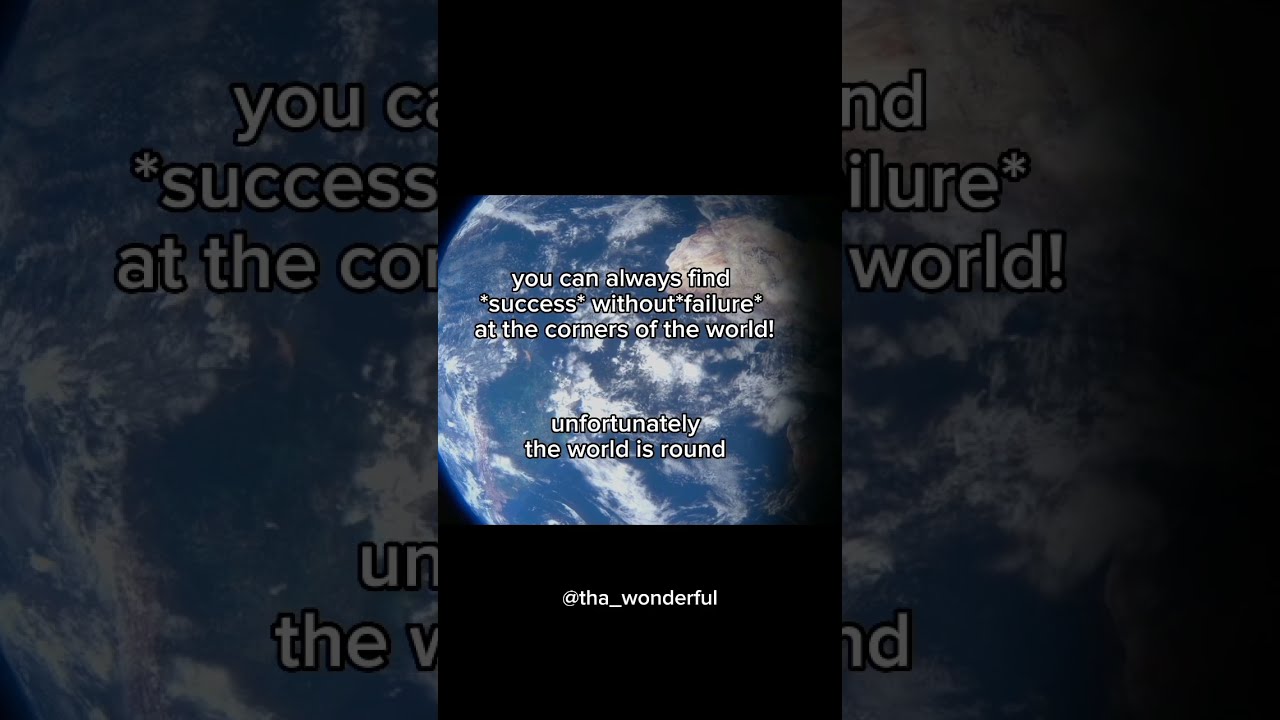This detailed image captures a sarcastic statement juxtaposed against a stunning view of Earth seen from space. The central portion of the image is dominated by a photorealistic depiction of our planet, showing a vibrant blue ocean, swirling white clouds, and a visible landmass off the coast of Africa. The poles of the Earth are cut off, focusing attention on the equatorial region. This central image is encased in a black border at both the top and bottom of the rectangular frame.

Overlaying the middle of the Earth image is a large, bold white text that reads: "You can always find *success* without *failure* at the corners of the world!" Below, it adds another line in smaller text: "Unfortunately, the world is round." This text conveys a witty, facetious commentary on the nature of success and failure.

The rectangular image appears to be a digital or poster design, possibly a social media post, as indicated by the Instagram handle "@tha_wonderful" in white text at the bottom black border. The background of the image is a larger, slightly blurred version of the same Earth photo, adding depth and framing the central content neatly. The overall design balances visual appeal with an ironic message, making it visually striking and thought-provoking.